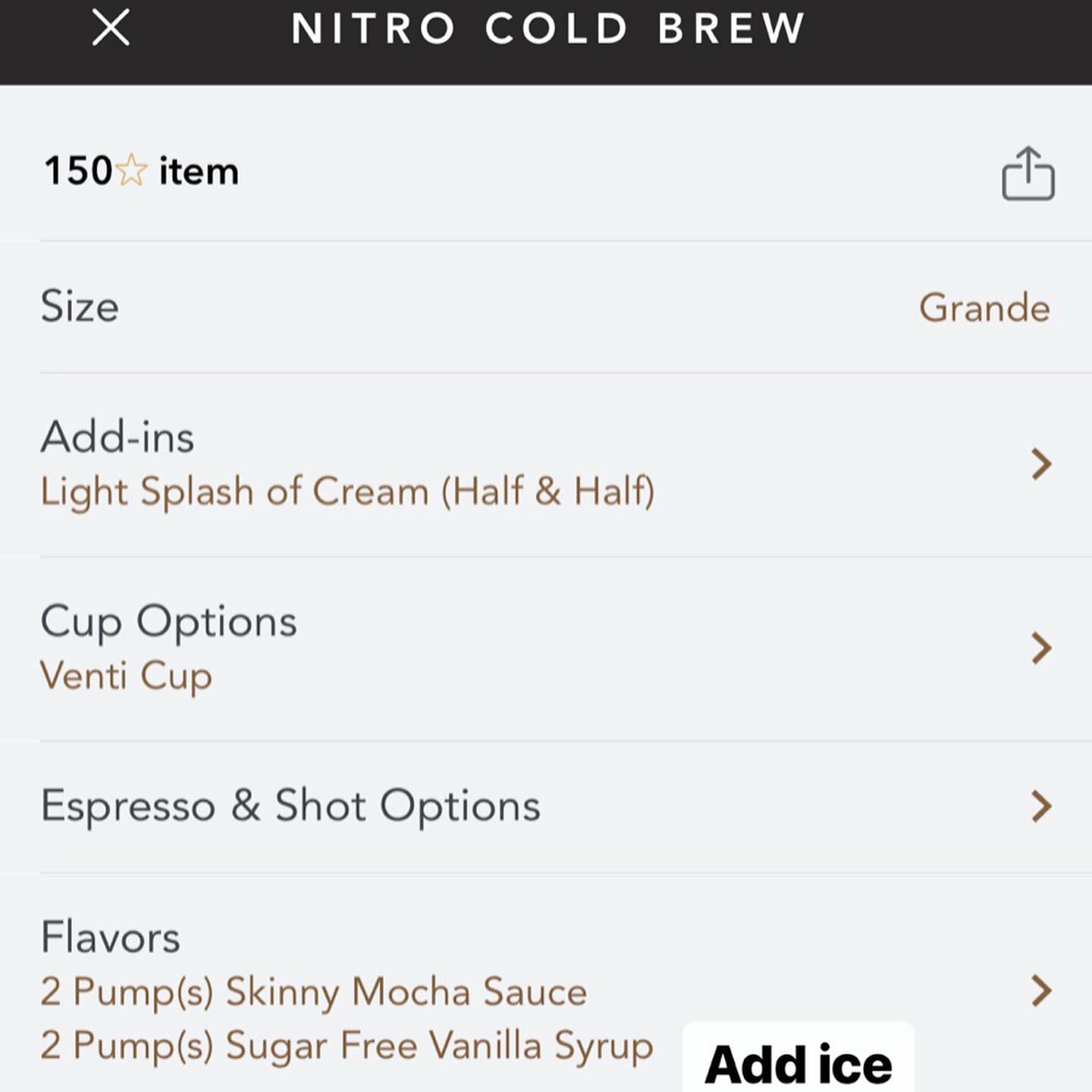Screenshot of a detailed coffee order from an unspecified location. At the top, "Nitro Cold Brew" is listed as the selected beverage, which is a 150-star item. The size chosen is "Grande." Under add-ins, there is a "Light splash of cream" with a specification for "Half and half." The cup size requested is "Venti." Espresso and shot options are mentioned, along with flavor customizations which include "Two pumps of skinny mocha sauce" and "Two pumps of sugar-free vanilla syrup." Finally, the order specifies to "Add ice." The image is entirely text-based with no photographic, illustrative elements, or any presence of people, animals, plants, vehicles, or other objects.